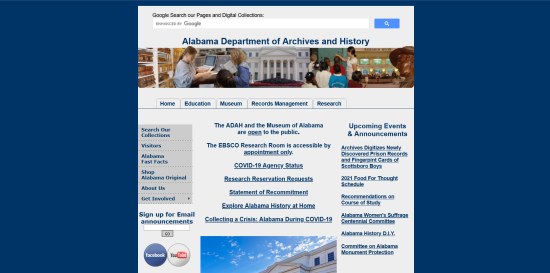The image presents a webpage surrounded by a blue border, with a thin navy blue line at the top and thick navy blue borders on the left and right sides. Central to the page is a Google search bar accompanied by the text: "Google search our pages and digital collections." Below the search bar, there is a blue search button with the text "Alabama Department of Archives and History" written in blue font.

Additionally, the webpage features images of a white building and several rooms where children are engaged in educational activities with teachers. Text below highlights various sections: "Home," "Education," "Museum," "Record Management," and "Research." It also states that the Alabama Department of Archives and History (ADAH) and the Museum of Alabama are open to the public, while noting that the Ibesco research room is accessible by appointment only.

Further informational sections include "COVID-19 agency status," "Research reservation requests," "Statement of Recommitment," "Explore Alabama history at home," and "Collecting a crisis: Alabama during COVID-19."